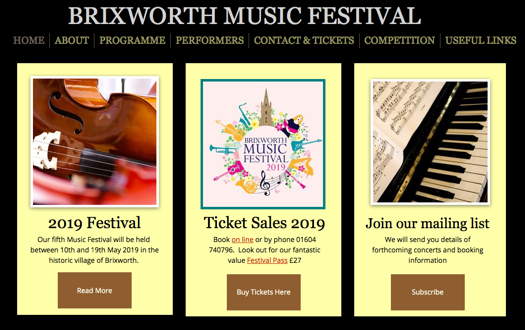This image displays a visually appealing website for the Bricksworth Music Festival. The header prominently features the festival's name, "Bricksworth Music Festival," in bold text, set against a pleasant yellow background. Just below the header, a navigation menu offers easy access to various sections: Home, About, Program, Performers, Contact, Tickets, Competition, and Useful Links.

The main content is divided into three distinct sections. The first section is titled "2019 Festival" and features a photograph of a cello, accompanied by text announcing that the fifth Bricksworth Music Festival will take place from May 10th to May 19th, 2019, in the historic village of Bricksworth. A "Read More" button, set in a brown box, invites users to explore further details.

The central section promotes the festival's ticket sales for 2019. It includes text encouraging attendees to book tickets online or by phone, and highlights the availability of a value-packed festival pass in red text. A brown box labeled "Buy Tickets Here" provides a direct link for purchasing tickets.

The third section calls for email list subscriptions. Featuring a picture of piano keys and part of a songbook with music notes, this section encourages visitors to join the mailing list to receive updates on forthcoming concerts and booking information. A brown "Subscribe" button is included for easy subscription.

Overall, the website offers a well-organized and inviting layout, effectively guiding visitors through the festival's offerings and encouraging engagement.